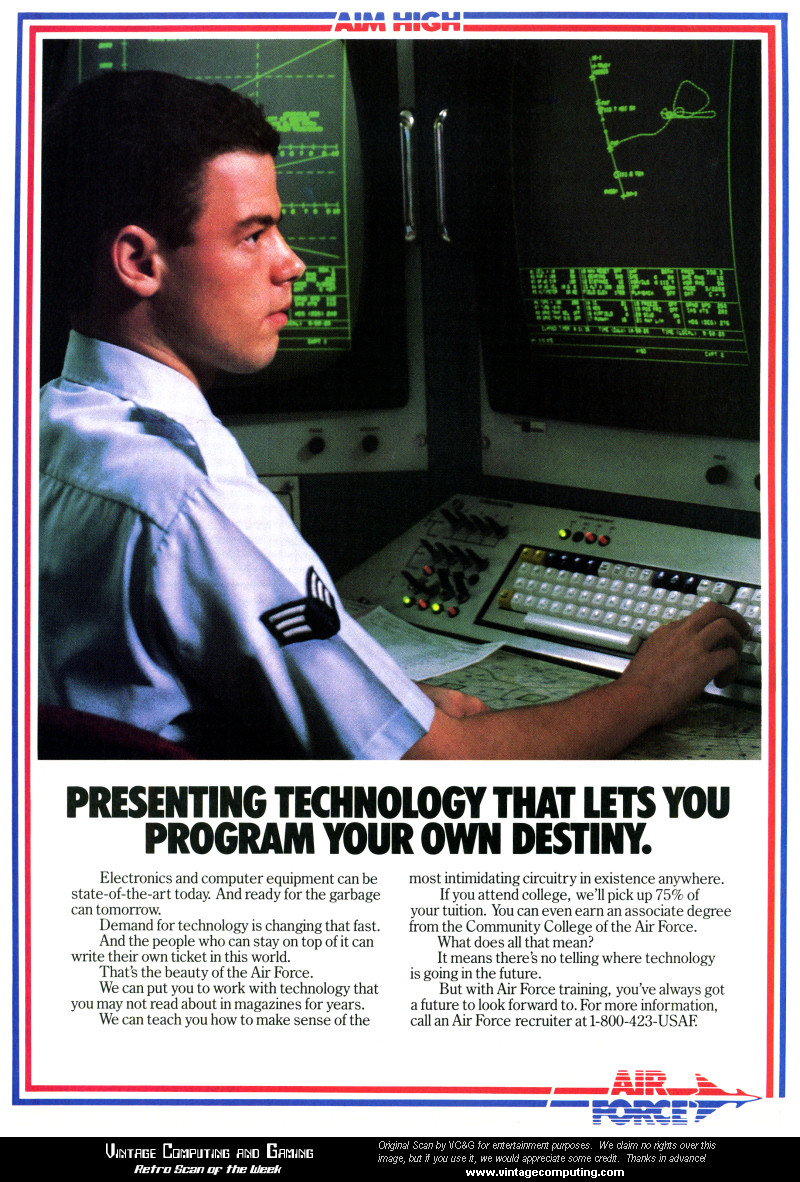This detailed caption consolidates shared and repeated details from all six descriptions, emphasizing the consistent elements to create a cohesive narrative:

This 1980s Air Force recruitment advertisement, likely from a magazine, presents a visually nostalgic combination of colors, fonts, and imagery from that era. The top of the ad reads "Aim High" in bold letters, with "Air Force" prominently placed at the bottom. The content is framed by a distinctive American-themed border consisting of red, white, and blue lines. Central to the image is a young Caucasian man, around 21 years old, dressed in a white short-sleeved Air Force uniform adorned with a crest on the right sleeve. He focuses intently on an old-fashioned computer setup, featuring a bulky keyboard and a classic black monitor with neon green text and diagrams. His right hand rests on the keyboard as he examines the data on the screen.

Underneath the image, a bold headline declares, "Presenting technology that lets you program your own destiny." The body text elaborates on the opportunities within the Air Force, emphasizing advanced technology and educational benefits. It reads: "Electronics and computer equipment can be state-of-the-art today and ready for the garbage tomorrow. Demand for technology is changing fast, and the people who can stay on top of it can write their own ticket in this world. That's the beauty of the Air Force. We can put you to work with technology that you may not read about in a magazine for years. We can teach you to make sense of the most intimidating circuitry in existence anywhere. If you attend college, we'll pick up 75% of your tuition. You can even earn an associate degree from the Community College of the Air Force. What does it all mean? It means there's no telling where technology is going in the future, but with Air Force training, you've always got a future to look forward to. For more information, call an Air Force recruiter at 1-800-423-USAF."

At the bottom right corner of the image, "Air Force" is inscribed in red and blue letters, accompanied by a small red, white, and blue airplane graphic. The ad is completed with a black bar that acknowledges the vintage nature of the scan and contains a website link for more information.